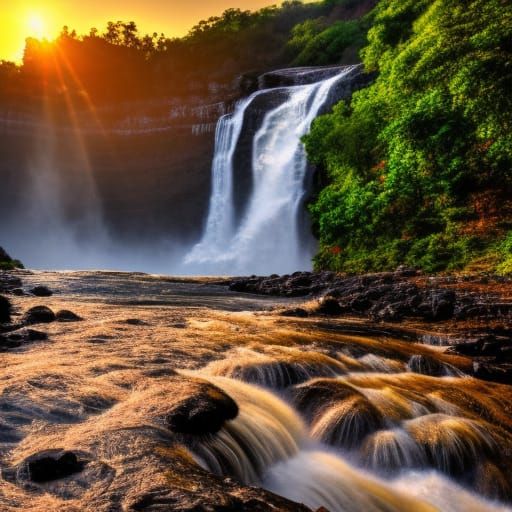This photograph captures a majestic and expansive waterfall cascading down a high cliff face, with vibrant white water streaming over the gray and darker-toned rocks. The waterfall, divided into two wide sheets, feeds into a swiftly moving river below, which flows with energetic white rapids and rocky shoals visible in the foreground. Lush, green vegetation, including trees and bushes, densely lines the cliffs and riverbanks, creating a stark contrast with the darker hues of the rocks and the river itself. An orange sun, possibly setting, beams its warm rays through the trees at the top left corner, casting a golden glow over the water and the surrounding landscape, enhancing the vibrant colors and adding a touch of serenity to the dynamic scene.